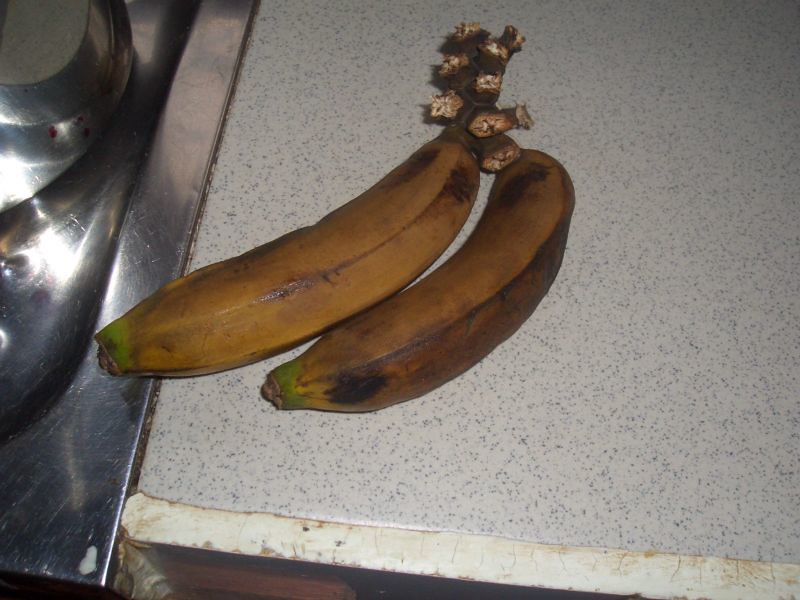A detailed view of a kitchen countertop reveals a distinctive design: a white surface marbled with black speckles stretches across the scene. To the left side, a stark contrast is created by a silver countertop, marked with numerous scratches indicative of frequent use. Overhead, a series of lights illuminate the area. The lower section of the image shows white cabinetry or trim, marred by stains and signs of dirt.

Prominently displayed on the left side of the countertop is an overly ripe banana, joined by another similarly aged banana on the right. The banana bunch atop has broken stems that reveal a white interior. The outer skins of the bananas are blotchy with black markings and show hints of green at the far ends. Dominantly brown, the bananas suggest they are nearing or have surpassed their peak ripeness stage, with much of their starch likely converted to sugar, making them very sweet. The scene, therefore, tells a story of a well-used kitchen space and the natural progression of produce stored within.